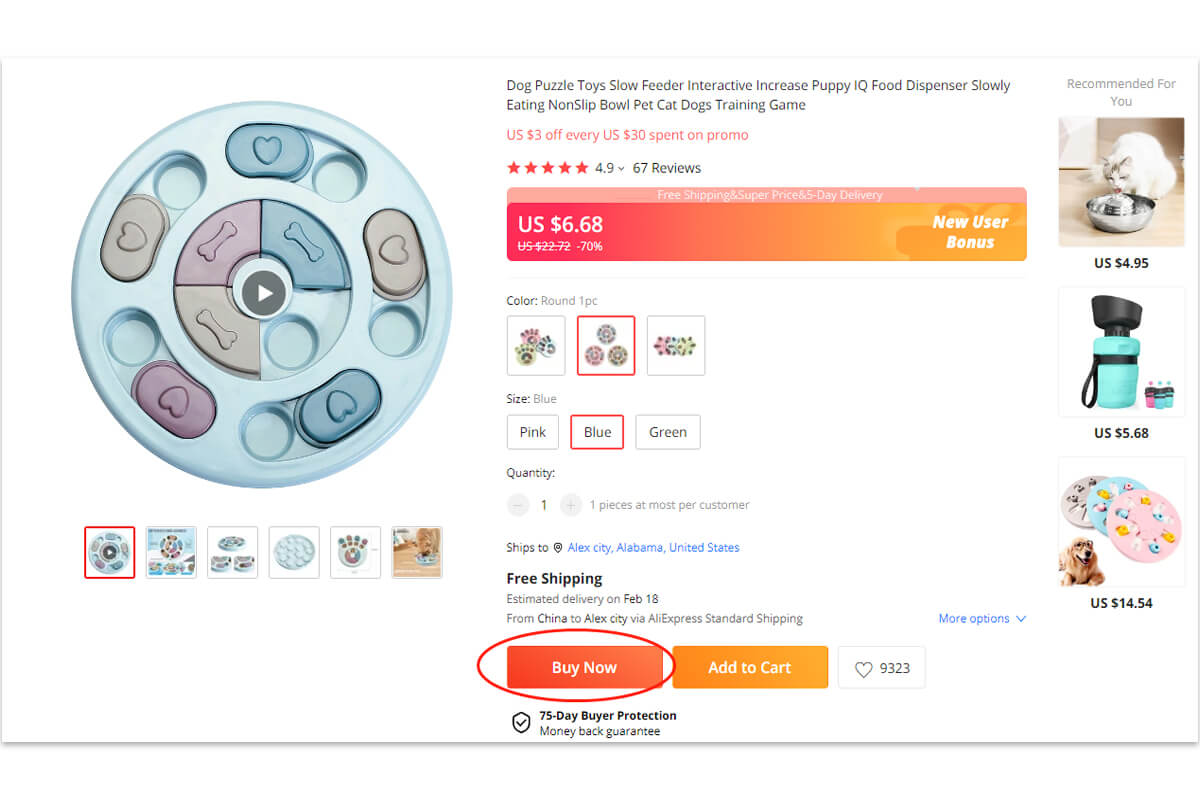Captured in the image is a comprehensive screenshot from an e-commerce website featuring a detailed product page for a pet item. The focal product is a "Dog Puzzle Toy Slow Feeder," designed to enhance puppy IQ and promote slow eating. This interactive food dispenser for cats and dogs showcases a vibrant image on the left, while the right side provides extensive product information.

The product boasts an impressive rating of 4.9 stars, as indicated by five red stars from 67 reviews. Beneath this rating, a prominent pink banner displays a discounted price: US $6.68, reduced from $22.72, reflecting a substantial 70% discount. Additional selling points noted include "Free Shipping," "Super Price," and "Five-Day Delivery."

Highlighted as a "New User Bonus," the page allows customers to select various options, including color and size, as well as the quantity. The currently chosen size is marked as blue, and the color option is "Round One PC." The header also emphasizes "Free Shipping." Key action buttons are styled distinctly – with a "Buy Now" button encircled in red, an "Add to Cart" button in orange, and a heart icon marked 9,323 times, presumably indicating user favorites or wishlist additions.

The product itself is a round feeder featuring dog bone and heart designs. It includes a compartment with a lid for placing food. Six high-quality studio photos, set against a white background, present multiple views of the feeder.

On the far right side of the screenshot is an "Ads Banner" section titled "Recommended for You," featuring related products: 
1. A stainless-steel water fountain for cats, priced at $4.95.
2. An aquamarine tumbler with a black cap, priced at $5.68.
3. A round dog toy available in various colors, priced at $14.54.

The detailed and organized layout provides a user-friendly experience for potential buyers.